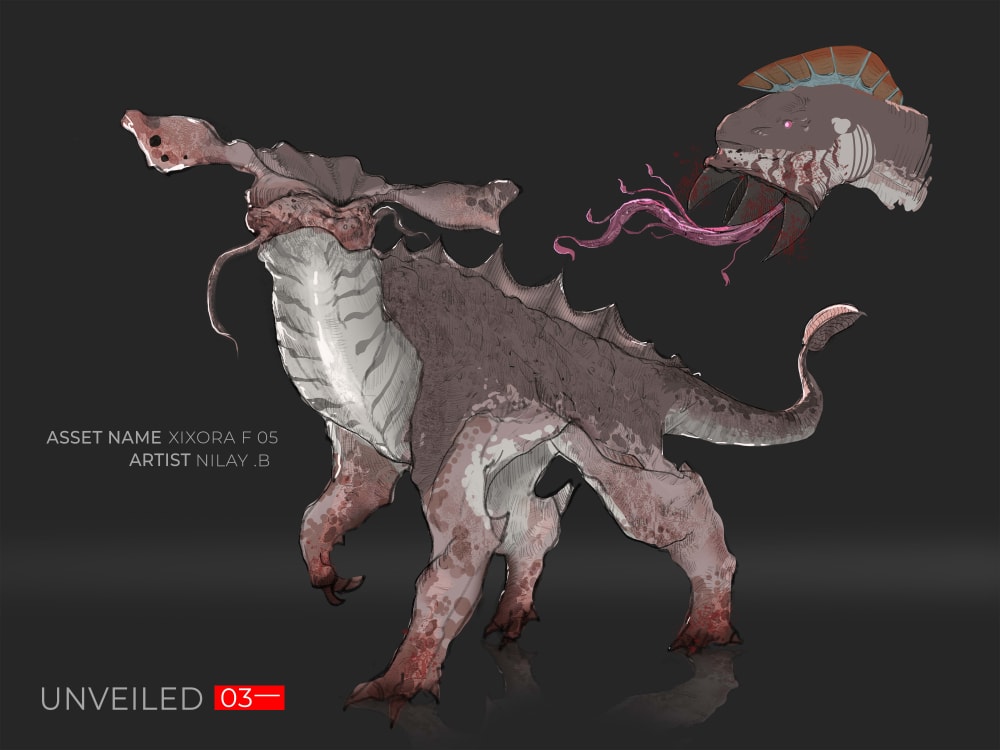The image depicts a computer-generated rendering of an intriguing creature set against a dark grey background. The focal point is a large, dinosaur-like entity positioned prominently on the right side. This creature features a distinct light brownish-purple hue, a massive tongue protruding from its mouth, and a grotesque, weird head. It has a bony underbelly, spikes adorning its back, and a substantial tail. Its eye is unnaturally extended to the side, and there are antenna-like appendages emerging from its mouth.

Accompanying this primary creature, on the left side of the image, you notice text that reads: "Asset Name: Csora 05, Artist: Nele B." At the bottom left corner, it states "Unveiled 03." Additionally, to the left of the main creature, there's another peculiar entity resembling an amoeba with a fin. This secondary creature appears almost mythical, with several antennae hanging from its lower body, enhancing the fantastical nature of the scene.